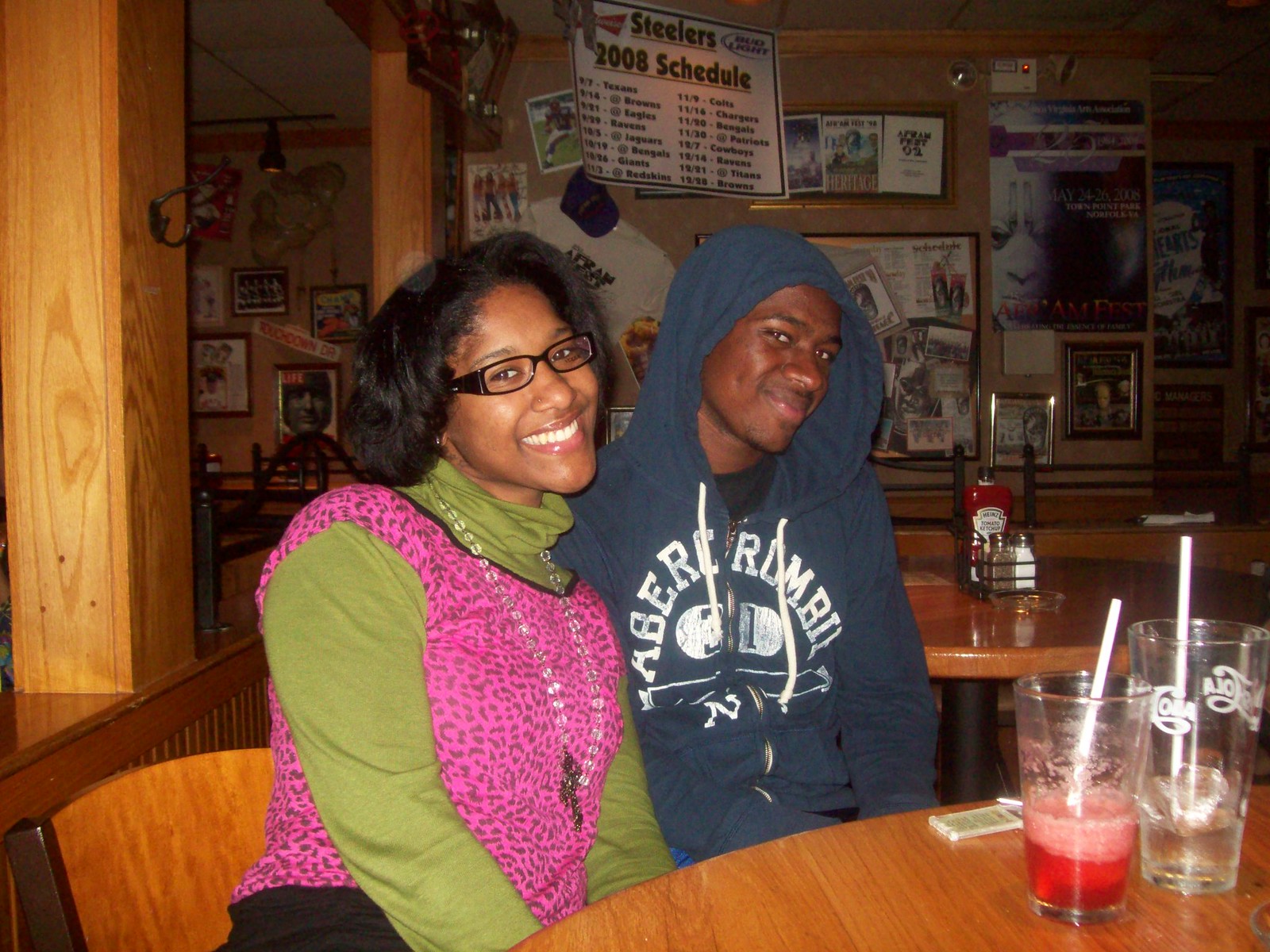The image features two African-American individuals seated at a light orange-colored wooden table in what appears to be a restaurant or bar. On the left is a woman with short black hair, wearing black glasses. She is dressed in a distinctive outfit that includes a green turtleneck under a pink cheetah-print top, paired with black pants. She is smiling warmly at the camera. To her right, and on the right side of the image, is a man wearing a blue Abercrombie hoodie, with the hood covering his head. The hoodie features the brand name in a circular white font. In front of them are two drinks: one is red, likely a soft drink, and the other appears to be water or Sprite. The table behind them holds condiments, including ketchup, salt, and pepper, and is identical to their own in its light orange hue. The background displays various posters and framed images, including a prominently featured Pittsburgh Steelers' 2008 schedule. They seem to be enjoying themselves and are posing for the camera, suggesting they might be on a date or having a good time out together. A wooden post and beams add to the rustic ambiance of the establishment.